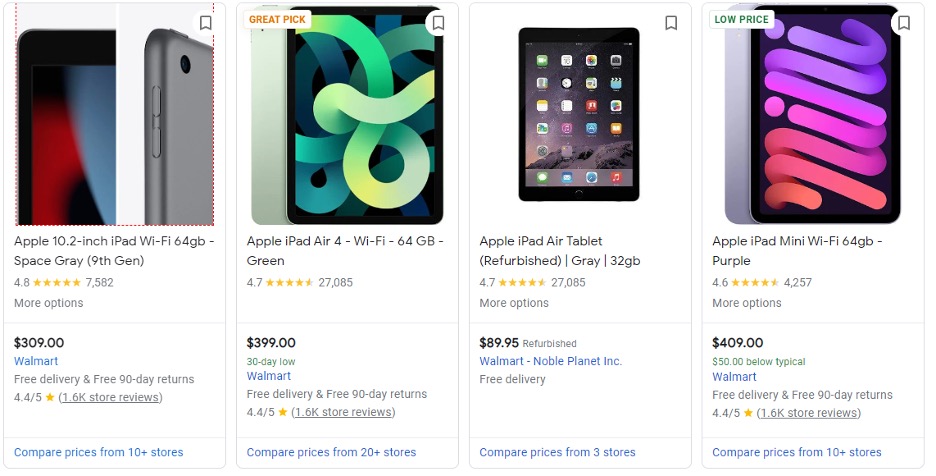In this image, we see a collection of four iPads listed as search results. The search engine displayed is not Google, indicated by the distinct font used. Each iPad is described with its specific details, prices, and ratings, all of which are available at Walmart and carry a 4.4-star review.

1. **Apple 10.2 inch iPad, Wi-Fi 64GB, Space Grey, 9th Gen** - Priced at $309.
2. **Apple iPad Air 4, Wi-Fi 64GB, Green** - Marked with a “Great Pick” label and priced at $399.
3. **Apple iPad Air Tablet, Refurbished, Grey, 32GB** - Priced at $89.95.
4. **Apple iPad Mini, Wi-Fi 64GB, Purple** - Highlighted with a “Low Price” label and priced at $409.